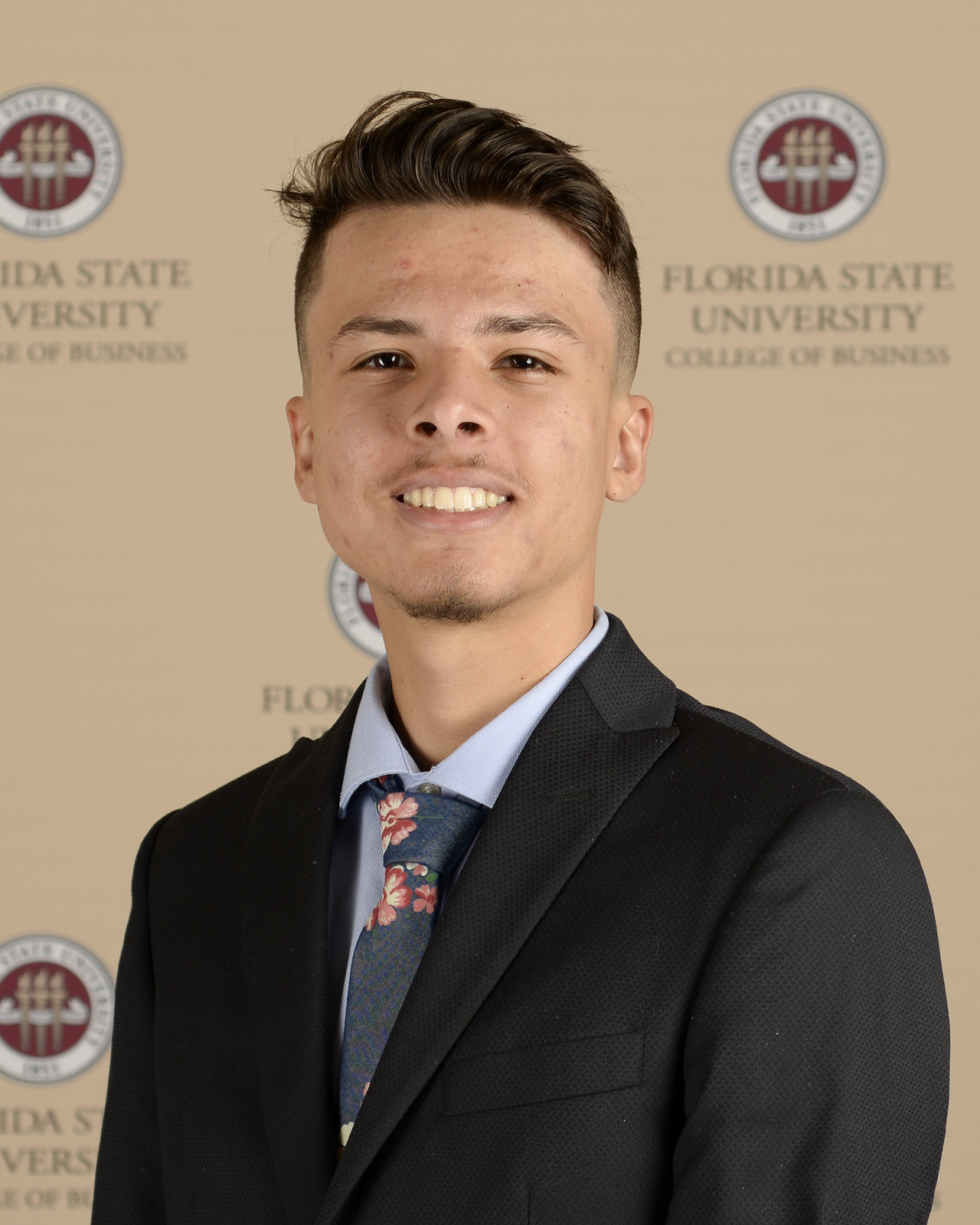The photograph features a young man, likely in his late teens or early 20s, smiling at the camera. He is dressed in a sharp, dark navy blazer (mistakenly referred to as black in one description), paired with a light blue collared shirt and a dark blue tie adorned with small pink or red flowers. His hair is distinctively styled, being longer and spiked at the top while shaved on the sides, contributing to a youthful appearance. He has light facial hair on his mustache and chin. The backdrop for the photo is a tan banner featuring the emblem and name of Florida State University College of Business in gray letters.